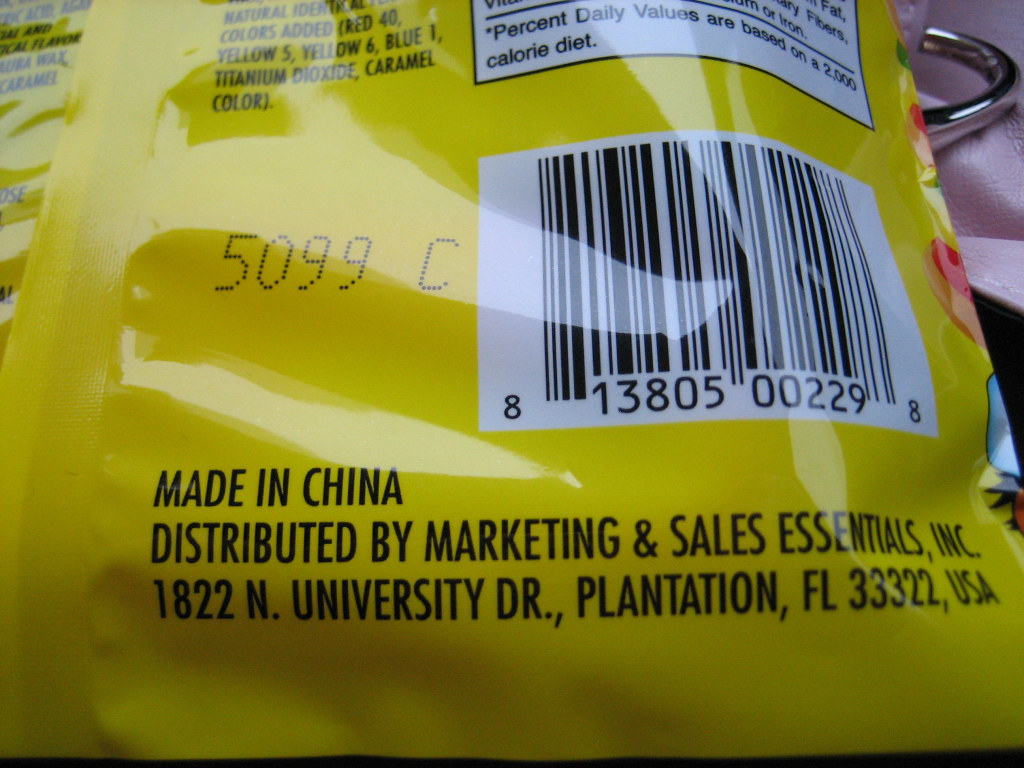This image displays the back of a yellow plastic food package. Prominently featured are the nutritional facts and ingredients list, though the latter is partially cut off. Ingredients listed include colors such as Red 40, Yellow 5, Yellow 6, Blue 1, titanium dioxide, and caramel color, suggesting that the package may contain candy. There is a mechanical printer code "0599C" visible, possibly indicating an expiration or production date. A white label above the barcode reads, "Percent daily values are based on a 2000 calorie diet." Below this, there is a UPC label with the code 813805002298. The text "Made in China, distributed by Marketing and Sales Essentials Inc., 1822 North University Drive, Plantation, Florida 33322 USA" is clearly printed. In the background, there seems to be a glimpse of a leather item, possibly a purse or a ring, and maybe a pair of scissors beneath the package, indicating that the photo was likely taken by someone to capture detailed information from the packaging. Additionally, the image faintly shows some print through the other side of the package.